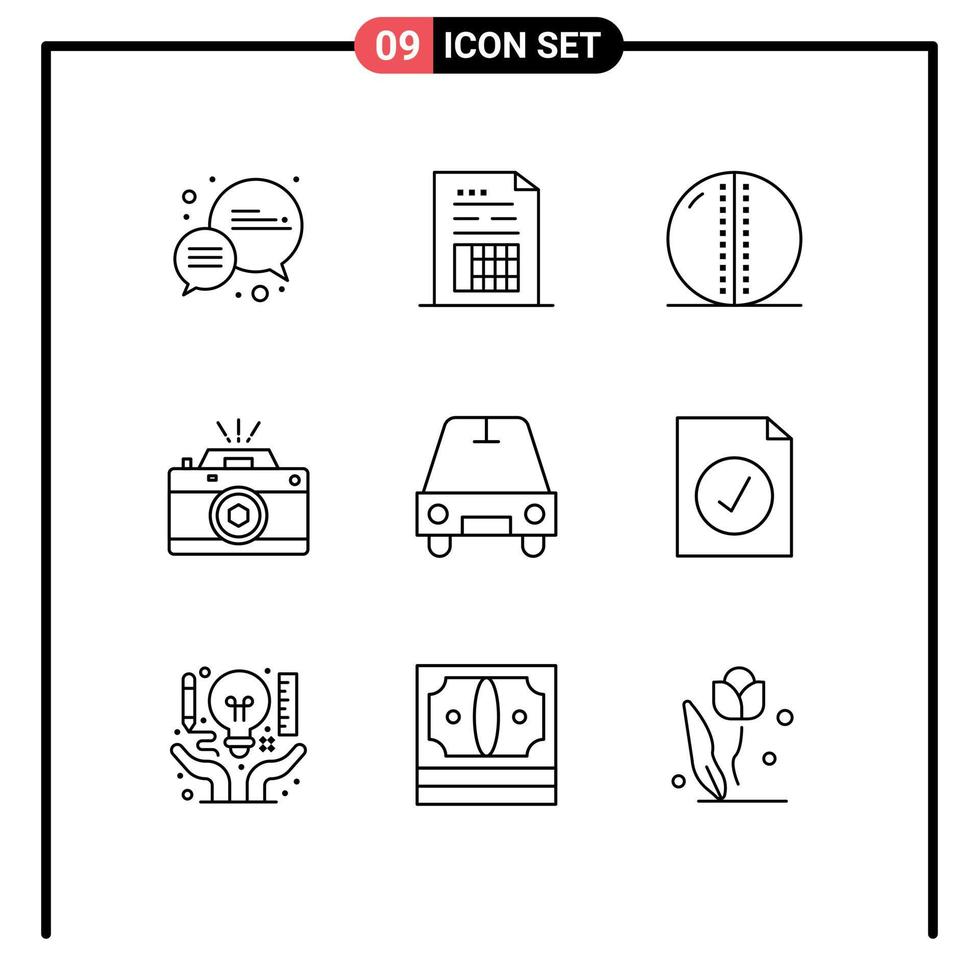This illustration features a black and white icon set titled "09" on a red background, with "icon set" in white font on a black background. Arranged in a 3x3 grid, the nine minimalist, simple line-drawn icons include: top left, text bubbles representing messages; top center, a graph or schematic; top right, a circle with a vertical line of squares; middle left, a camera icon; middle center, a car; middle right, a sheet of paper with a check mark, indicating a checklist; bottom left, hands holding a light bulb, ruler, and pencil, symbolizing inspiration and creativity; bottom center, possibly a theater ticket; and bottom right, a flower or rose. The arrangement and styling give it the appearance of icons possibly intended for a user interface or illustrative guide.